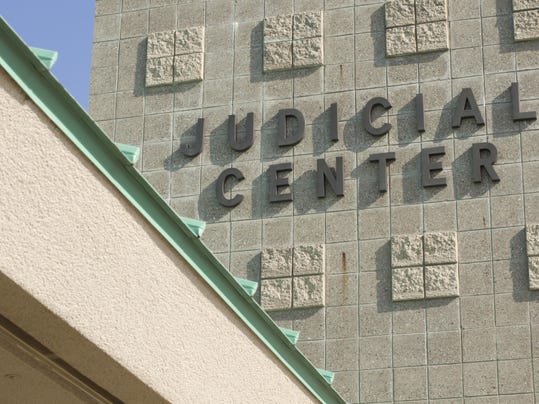The image captures a stone building prominently displaying "Judicial Center" in large, dark brown letters. The walls of the building are composed of symmetrically arranged square tiles, forming a uniform grid pattern. Notably, clusters of four tiles come together to create larger squares positioned above and below the central "Judicial Center" lettering. The lower left corner reveals a portion of a nearby roof, characterized by its light green metal surface and cream-colored edges. A sliver of clear, blue sky is visible in the top left corner of the frame. The day seems sunny, as indicated by the shadows cast on the left side of each letter, suggesting that the sun is shining from the right side of the image.